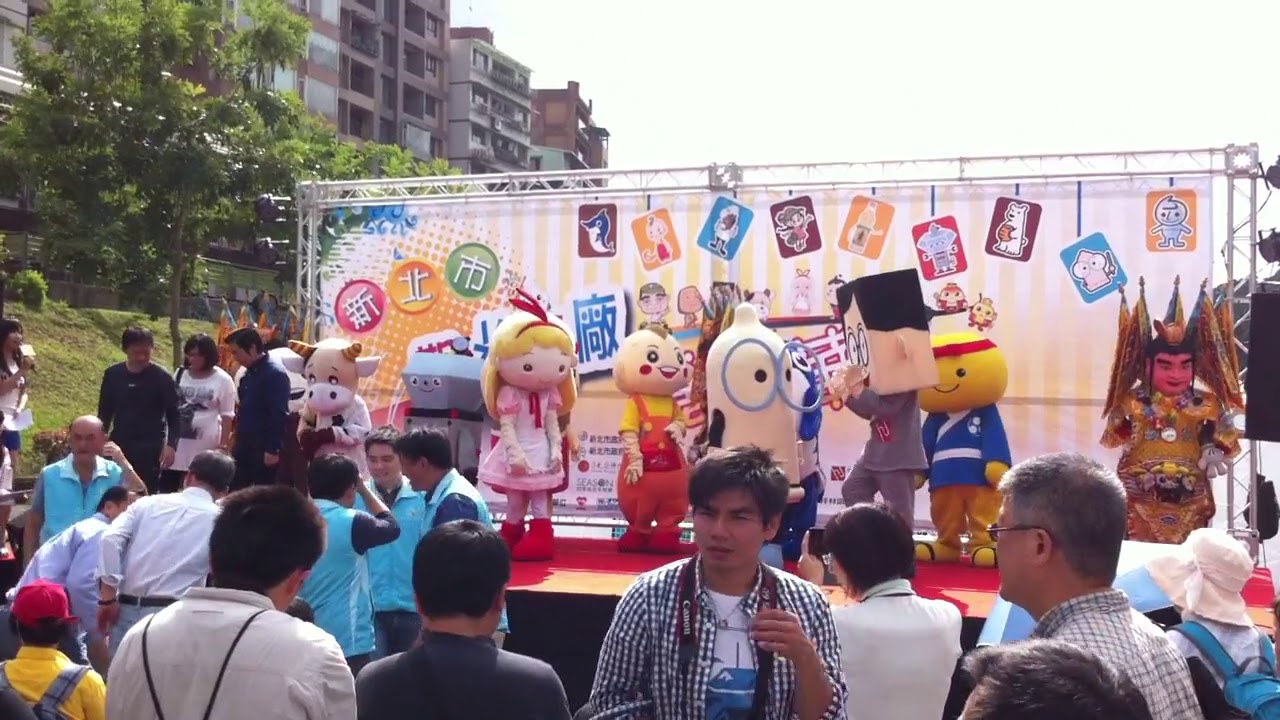The image depicts a bustling outdoor scene centered around a vibrant stage, set against a backdrop of urban buildings and natural elements. On the left-hand side of the picture, a gentle hillside with sparse trees ascends towards a cluster of multi-story apartment buildings. The sky, clear with a sharp glare, subtly lights the entire setting. Positioned at the base of the hillside and extending towards the center of the image is a congregation of people, their backs primarily turned towards us, capturing the viewer's focus on the stage.

The stage, a short platform with a red floor, is framed by a sturdy metal structure that supports a large, colorful banner adorned with Japanese characters and various animated figures on a yellow and white striped background. The stage itself hosts a collection of costumed characters. From left to right, these include a cow, a robot with a hexagonal head and a smiling face, a girl in a pink dress, a baby in an orange jumpsuit, a dome-headed character with large round glasses, a man with a square head in a gray suit, and a yellow-headed figure with a red headband. On the far right stands an elaborate character with a golden outfit and an ornate headdress.

In front of the stage, the crowd is dynamic, with several men equipped with cameras, some wearing flannel shirts and hats, evidently capturing the event. Highlighted in the foreground are three individuals, one of whom wears a polka-dotted shirt and faces slightly left. Beside him is a man with glasses and short hair facing left, with other indistinguishable people nearby. Along the left edge of the image, a few people are seen walking toward the main crowd, adding to the lively atmosphere of this eventful scene.